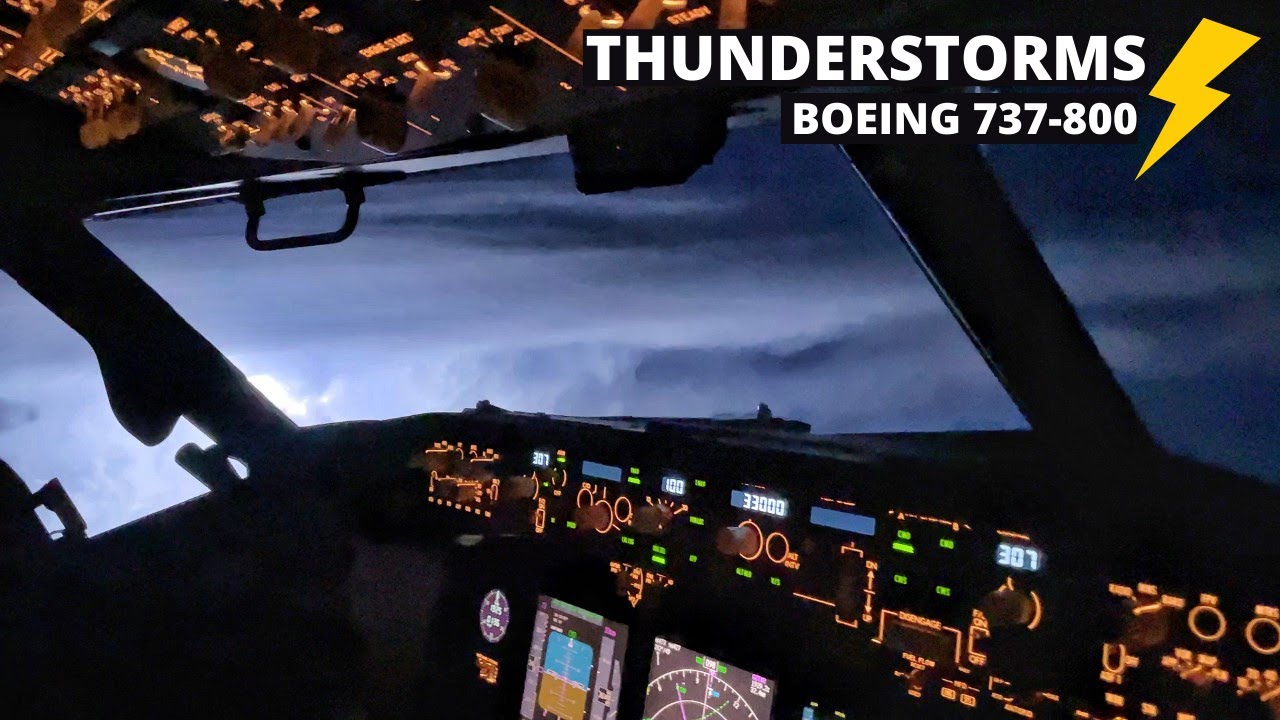This detailed color photograph captures the intricate cockpit of a Boeing 737-800 jet in flight. The illuminated control panel is prominently featured, showcasing a myriad of screens, dials, and instruments essential for navigation and aircraft control. Through the expansive windshield, fluffy clouds accompany a deep blue sky, hinting at a serene yet dynamic atmospheric scene. Overhead, the ceiling lights add a subtle glow to the sophisticated cockpit environment. Notably, the image bears a striking caption in bold, all-caps white lettering situated in the top right corner, which reads "THUNDERSTORMS Boeing 737-800" alongside a vivid icon of a yellow lightning bolt. This composition, wider than it is tall, is devoid of any people, animals, plants, flowers, trees, or automobiles, focusing entirely on the advanced avionics and serene sky outside.